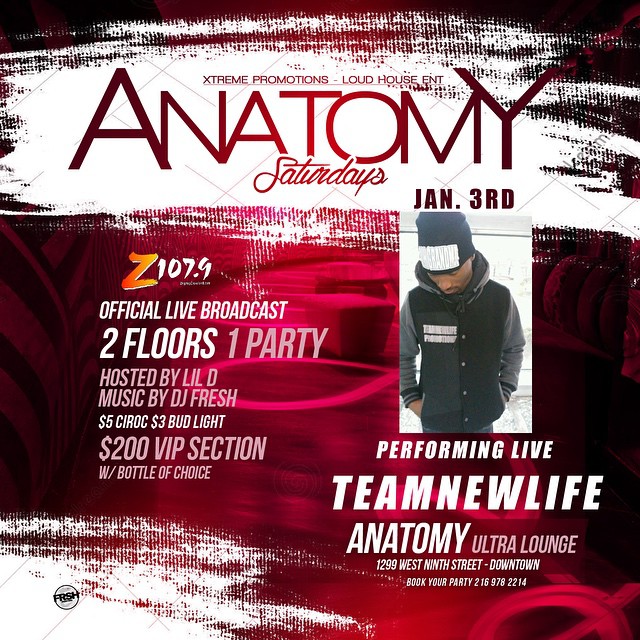The flyer is a promotional piece for an event hosted by Extreme Promotions and Loud House Entertainment, taking place on January 3rd at the Anatomy Ultra Lounge. The design features a predominantly red background with white paint strokes across the top and bottom, giving it a striking visual contrast. Prominently, "Anatomy Saturdays" is written in large print with a gradient effect transitioning from bright red to a darker shade towards the edges. 

On the left side of the flyer, "Z107.9 Official Live Broadcast" is displayed in bold letters, followed by event details such as "Two Floors, One Party, Hosted by Lil D" with music by DJ Fresh. Drink specials include $5 Ciroc and $3 Bud Light, with a $200 VIP section offering a bottle of choice. 

In the lower left corner, there's a black circle bearing the "FRSH" logo. To the right side of the flyer is a photograph of an African American man wearing a black beanie and a black and gray jacket with a hood. Beneath his photo, the text reads: "Performing Live, Team New Life, Anatomy Ultra Lounge, 1299 West 9th Street, Downtown. Book Your Party: 216-978-2214." The flyer effectively combines vibrant colors and detailed event information to draw the viewer's attention.